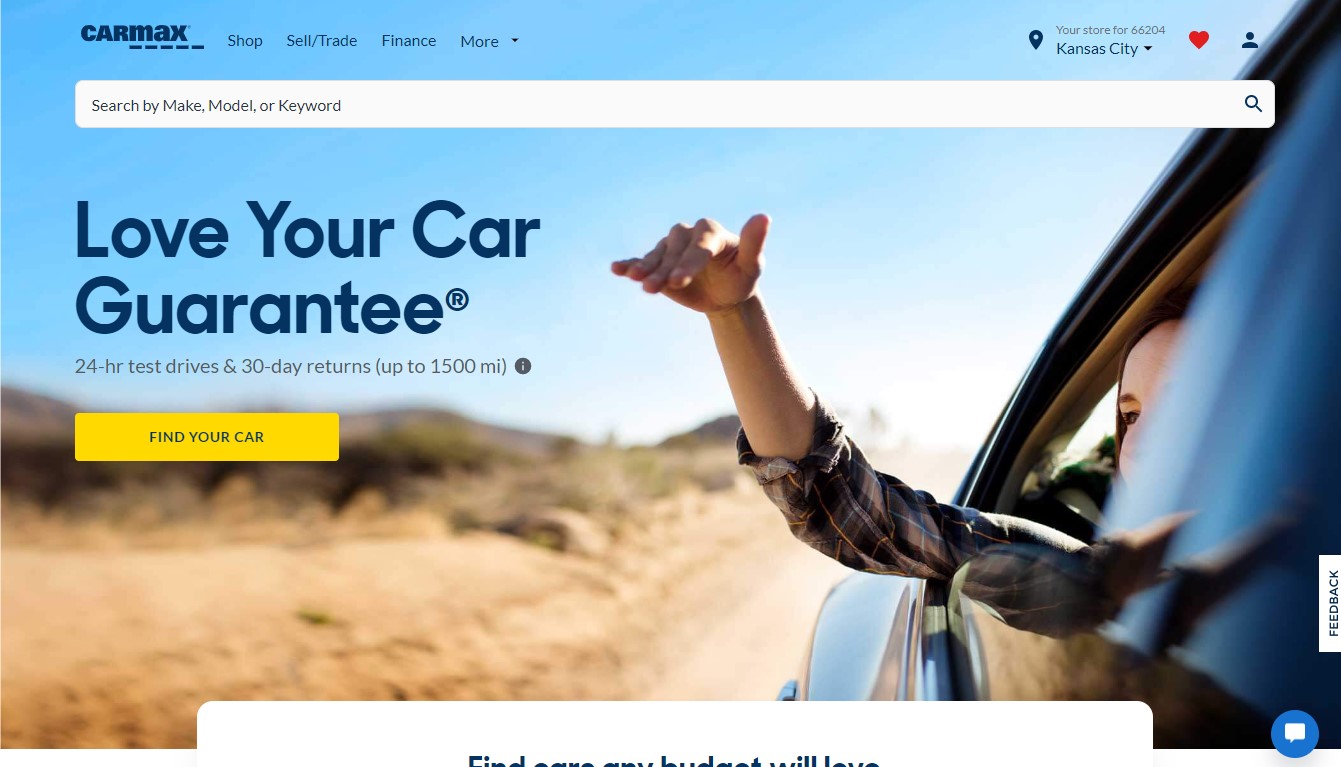The home page of the CarMax website prominently features the CarMax logo in the upper left corner. The webpage greets visitors with a large hero image that captures a vibrant scene: a young female, likely from the backseat on the passenger side, has her hand extended out the window. She's wearing a plaid flannel shirt with rolled-up sleeves. Her hand is flat against the air, as if she's surfing the air pressure created by the moving car. The car itself blurs in the foreground due to a tight, shallow depth of field, while the background features a picturesque landscape with dirt on the roadside, a blend of brown and light green shrubs, and rolling hills against the horizon.

Adjacent to the CarMax logo are navigational options including "shop," "sell," "trade," "finance," "more," followed by a location marker indicating "your store 466204 in Kansas City," and icons for favorites (heart) and user profile. A large search field is provided, allowing users to search by make, model, or keyword.

Overlaid on the hero image, bold blue text reads "Love Your Car Guarantee," featuring two key benefits: "24-hour test drive" and "30-day returns up to 1,500 miles." Below this text, a prominent yellow button invites users to "Find Your Car." At the bottom of the page, partially visible text on a white rectangle suggests phrases like "find cars any budget will love," though the full text is slightly obscured.